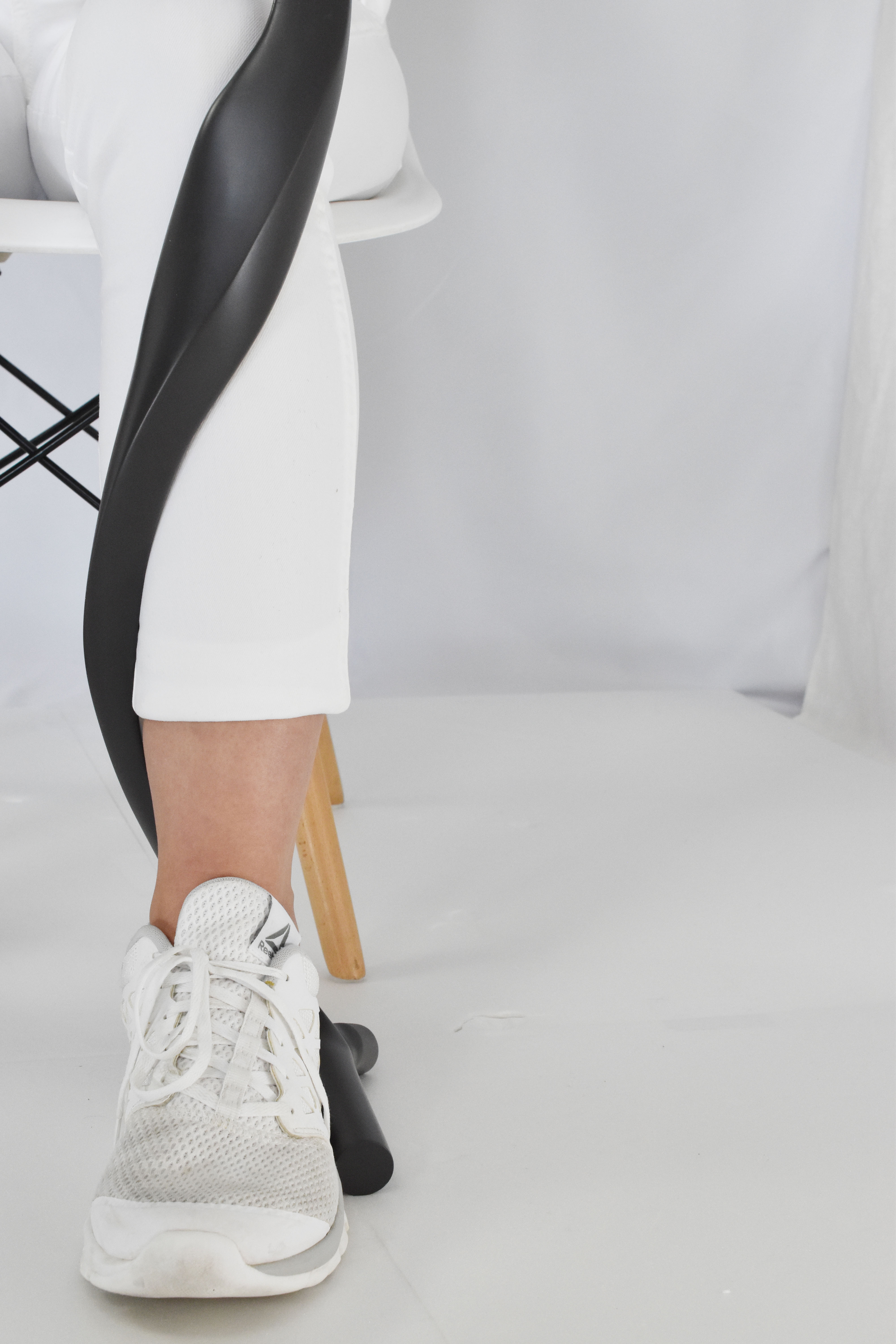This image features a close-up of a woman's leg, visible from the knee down, as she sits in a chair. Her leg is intertwined with a shiny black, twisted metal bar, which appears to wrap around her limb from mid-calf to ankle, almost like the leg of the chair itself. The woman is wearing white ankle pants and white Reebok tennis shoes with white shoelaces. The chair she is seated on has a white seat with light brown wooden legs, featuring a black metal frame beneath it. The background is predominantly white, including the floor and curtains, adding to the overall monochromatic theme of the setting.